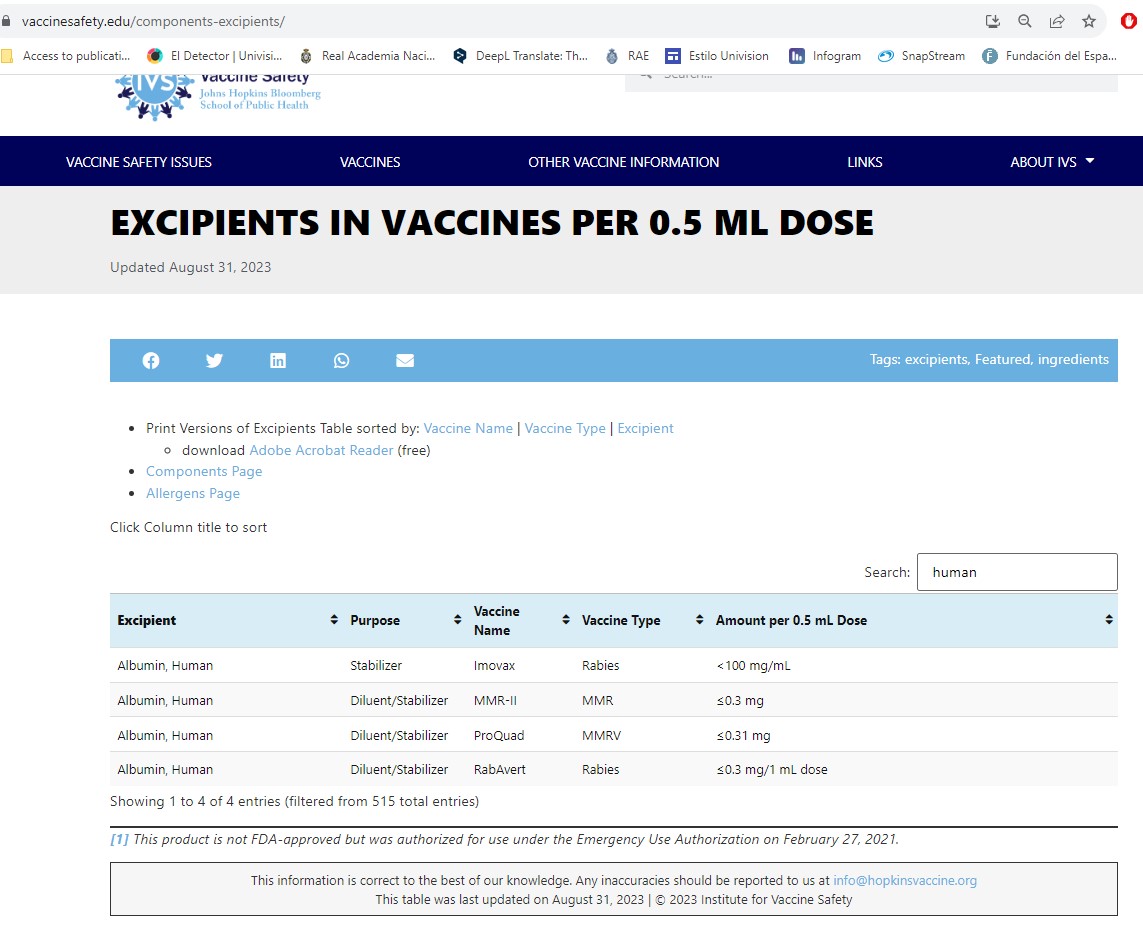The image showcases a screenshot from the website "vaccinesafety.edu," which appears to be an educational platform, possibly affiliated with a university. The logo indicates that it belongs to the "Vaccine Safety" initiative of the Johns Hopkins Bloomberg School of Public Health, lending it an official and credible status. The top section of the webpage includes various navigational links such as "Vaccine Safety Issues," "Vaccines," "Other Vaccine Information," "Links," and "About IVS."

The title displayed on this particular page is "Excipients in Vaccines per 0.5 Milliliter Dose," with "excipients" being explicitly spelled out. Notably, the information was last updated on August 31, 2023. The main content features a detailed table listing various excipients found in vaccines. The table is organized into several columns, including "Excipients," "Purpose," "Vaccine Name," "Vaccine Type," and "Amount per 0.5 Milliliter Dose." While the excipients remain consistent across the entries, the purposes, vaccine names, types, and amounts vary.